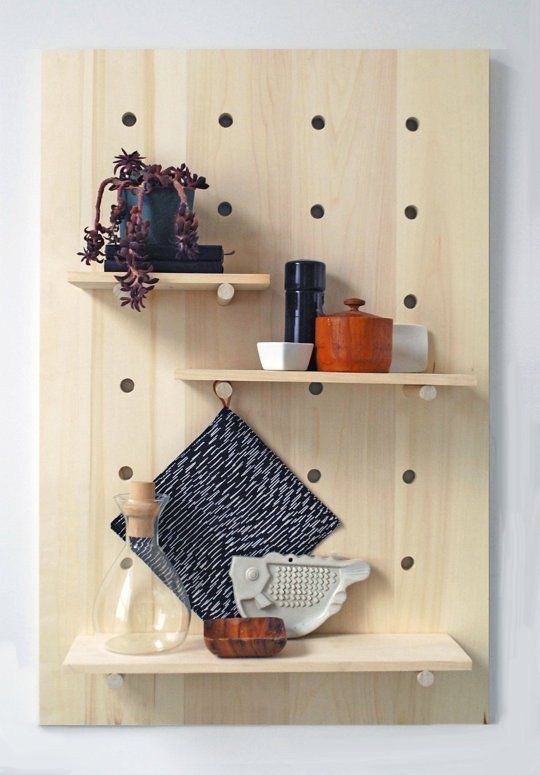The image depicts a light brown rectangular wooden board mounted vertically on a white wall. The board is designed with a grid pattern of seven rows of four holes each, allowing for the adjustable placement of shelves. Three shelves are currently attached to this board using wooden dowels inserted into the holes. 

The uppermost shelf, positioned on the top left, holds a blue pot with cascading purple flowers. The middle shelf, situated more to the right, includes an assortment of containers: a white bowl, a black cylindrical container likely used for spices, a red terracotta pot with a lid, and another white container adjacent to it. The bottom shelf, which spans the full width of the wooden board, houses a clear flask with a cork stopper, a piece of blue and black diamond-shaped fabric, a white fish-shaped object, and a small wooden bowl. This comprehensive setup creates an organized display of various household items against a clean, white background.